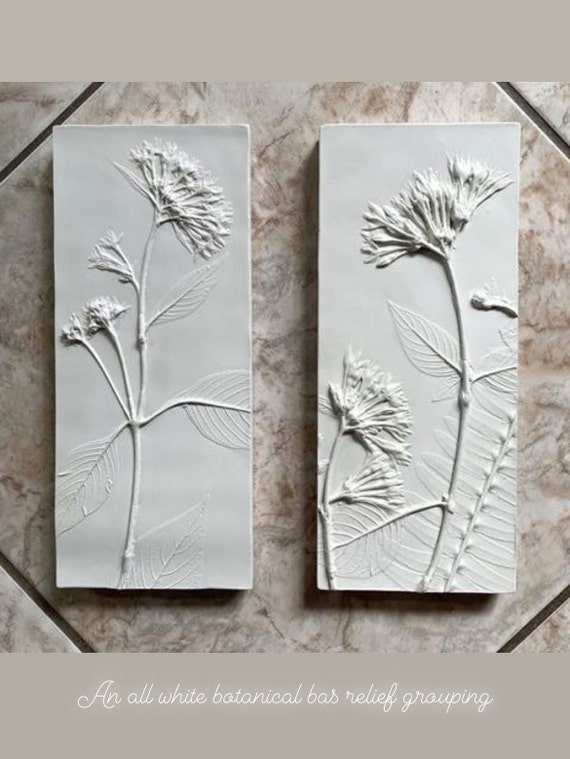The image depicts two tall rectangular bas-relief sculptures, perfectly centered on a large ceramic tile with a marble-like texture. Both sculptures showcase botanical motifs, specifically flowers carved with intricate details in white stone or clay, creating an all-white botanical bas-relief grouping. The left-hand sculpture features a main flower with four buds and three leaves emanating from a primary stem, while the right-hand sculpture shows two main stems – one producing a single large flower and the other with two smaller blooms and several leaves. The carvings, though similar in theme, differ in their floral arrangements, mimicking natural variations. The background tile resembles a kitchen floor, reinforcing the sculptures' placement and emphasizing their aesthetic contrast against the beige backdrop.